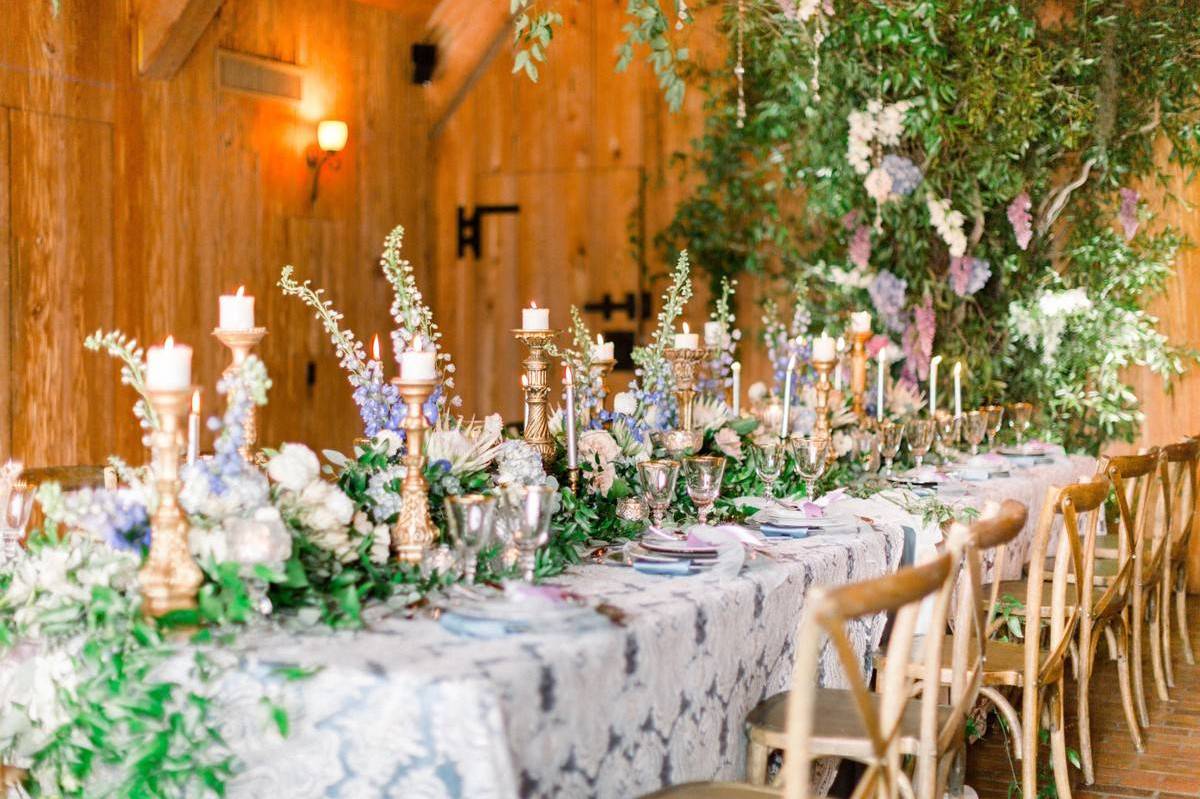This landscape-oriented photograph captures a beautifully decorated long table, likely set for a wedding reception. The table extends from the bottom left to the center right of the image and is adorned with an elegant white and light blue lace tablecloth. A lavish array of centerpieces runs down the entire length of the table, featuring abundant greenery and floral arrangements, some with lavender, intertwined with gold candelabras holding white candles. These lush decorations nearly obscure the place settings, which include plates and gold-rimmed glasses meticulously arranged at each seat. The table is surrounded by wooden or gold-toned chairs, with five clearly visible on the right side. In the background, the room's ambiance is enhanced by rich wood paneling, reminiscent of a barn, and additional greenery climbing the far wall, complementing the forest-like decor at the table's end.